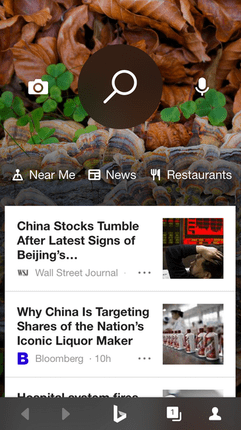The image presents a multi-layered collage featuring a variety of elements. The top section consists of what appear to be brown leaves and green shamrocks, accompanied by beige, gray, and bronze rocks or seashells. On the left side of a central black circle, a white camera icon is visible, while on the right side, there is a white microphone icon. Inside the circle itself is a white magnifying glass. Spanning across what seems to be the rocks or seashells are white text labels that read "near me," "news," and "restaurant" (with a fork and knife icon next to it).

Below this, there is a rectangular-shaped pop-up with its bottom cut off. This pop-up has a predominantly white background with a black header. The first line of text reads "China stocks tumble," followed by "the latest signs of" on the next line, and then partially visible text "Beijing's..." ending in an ellipsis. Immediately below, the letters "WSJ" are in a darker font, with "Wall Street Journal" in gray beneath it.

Continuing downward, there is an image of a man, where only his head and arm are visible. He is wearing a black shirt and appears stressed as he looks at red charts. A thin gray line runs across this section with the following black text: "Why China is targeting" on one line, "shares of the nation's" on the next, and "iconic liquor maker" on the last. A purple bead icon is also present, accompanied by the text "Bloomberg" in gray and a timestamp indicating "10H ago." Another set of three black plus signs is visible at the bottom of this section.